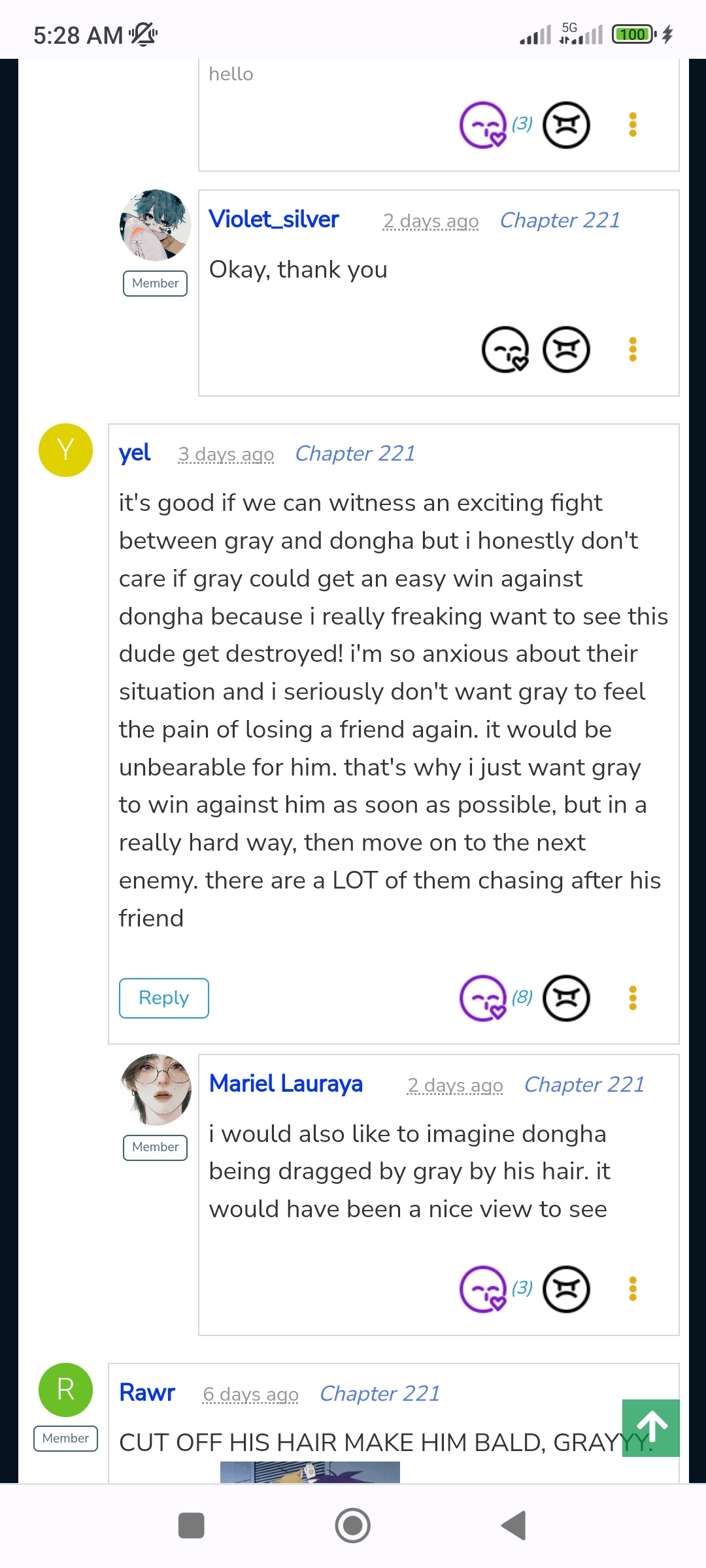Screenshot of a mobile device displaying a review website. The app interface showcases a community discussion with comments, upvotes, and downvotes. Prominently, a user under the handle "Violet_Silver" posted two days ago about witnessing some sort of altercation, prompting a heated exchange among multiple users. Usernames are highlighted in bold, with options to react to comments using smiley or unhappy faces. Various topics populate the screen along with user avatars in vibrant violet and blue tones. Notably, the discussion appears under "Chapter 221," though the specific subject of the argument remains unclear.